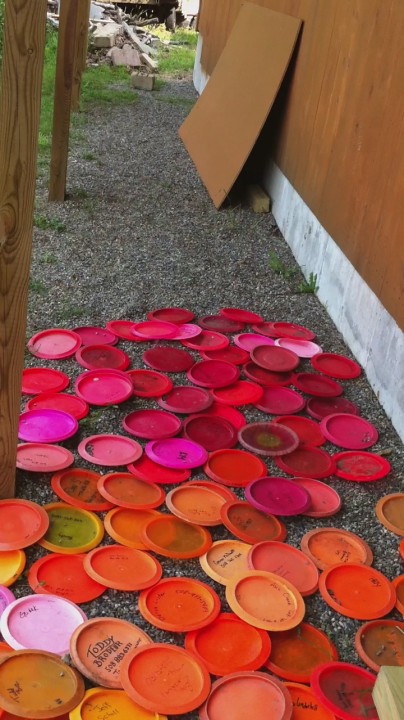In this outdoor photo, a gravel walkway sits in front of a wooden fence that's built atop a short concrete wall, creating a rustic backdrop. To the right, a piece of wood or cardboard leans against the wall, adding to the scene's casual disarray. The main focus is an assortment of disc golf frisbees scattered across the gravel walkway. These frisbees are sorted by color, transitioning from orange at the bottom of the image, to pink in the middle, and red towards the top. Some of these frisbees have small, unreadable writings on them. In the background, there's a distant view of grass dotted with various debris, suggesting abandonment or disorder. Additionally, two wooden beams or supports emerge from the ground, likely part of a structure. This detailed arrangement captures a sense of neglect mixed with vivid, haphazard organization.